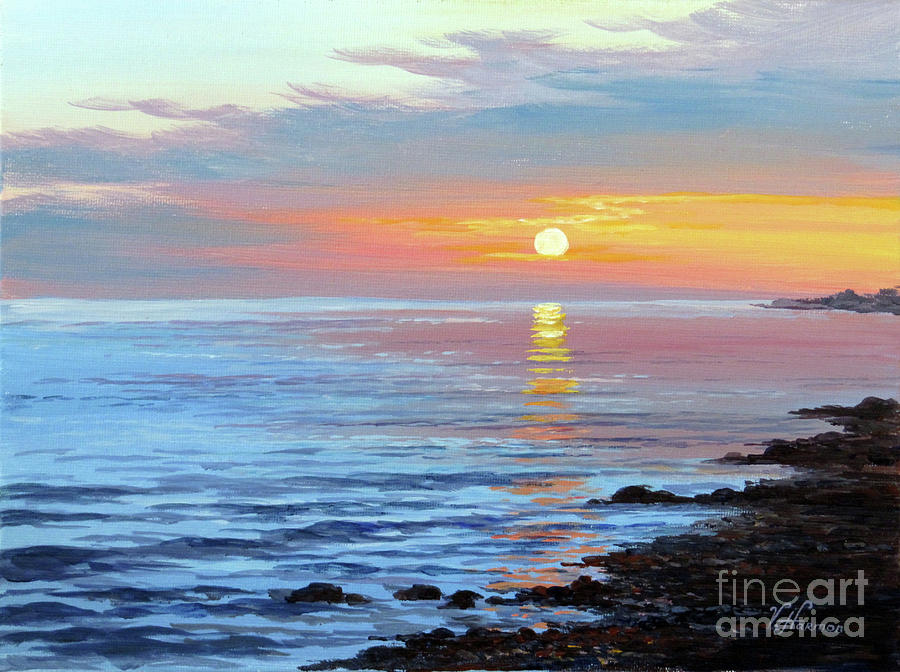We are looking at a fine art painting of a sunset over a large body of water, with the scene likely captured along a rocky seashore. The horizon is tinged with vibrant colors as the sun, glowing a rich orange, appears to descend into the water. The sky in the upper left-hand corner is a clear light blue, transitioning to wispy clouds that gather and become densely orange and yellow as they approach the sun's position towards the center of the image. These clouds blend into darker red and blue hues on the right-hand side, creating a dramatic contrast. The water is fairly still, depicting subtle ripples that perfectly mirror the contrasting sky above. Beneath the reflection, a golden strip of sunlight extends toward the forefront of the scene. The shoreline at the bottom right-hand corner is covered with dark gray rocks, indicative of a rugged seashore. A small peninsula juts out towards the center right of the painting. In the bottom right-hand corner, the white lettering "Fine Art America" is visible, suggesting the painting is available for purchase.